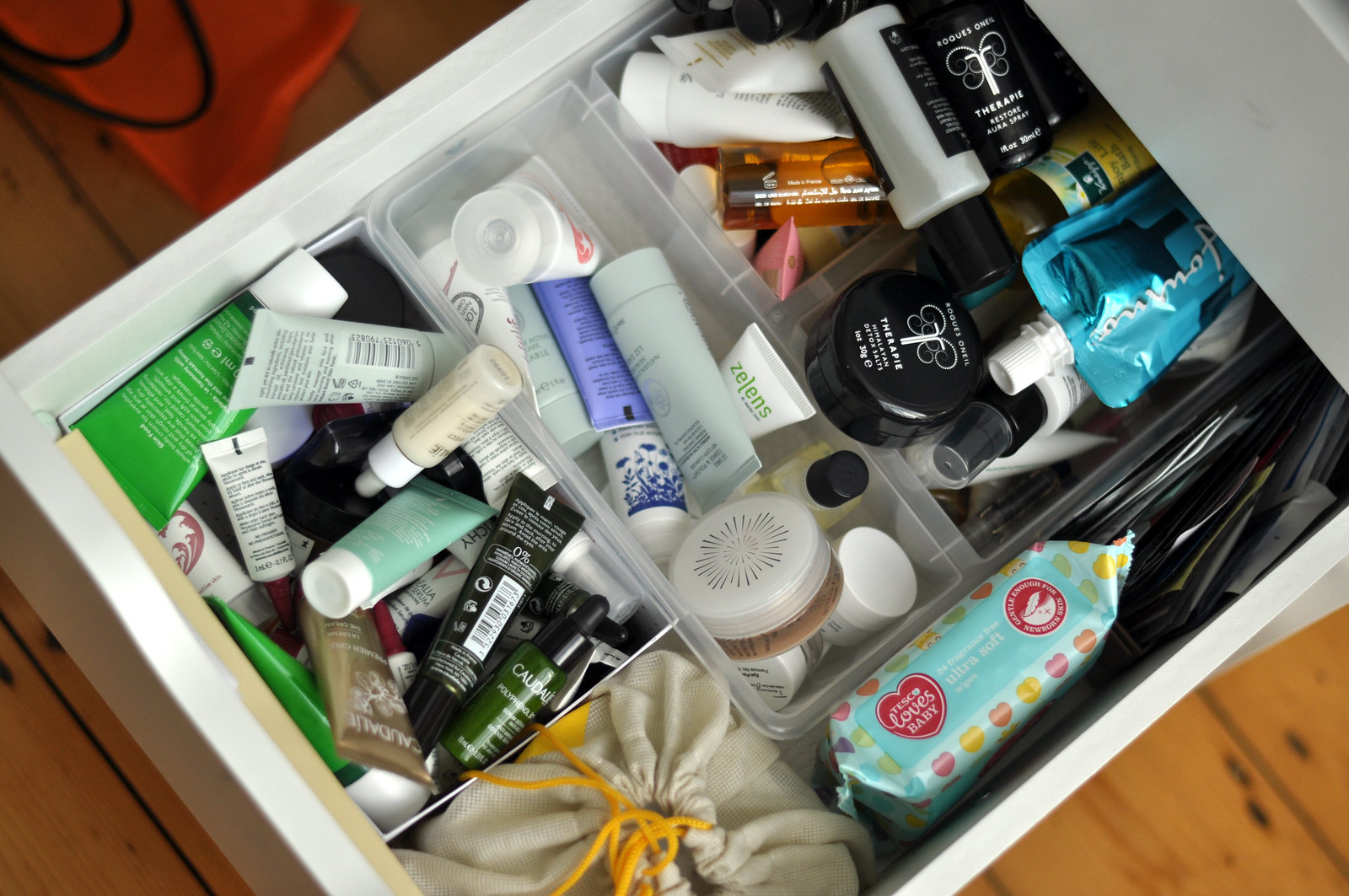The image is a detailed top-down view of a makeup or beauty supply drawer positioned over a light brown laminate wood panel flooring with visible dark knots. At the top edge of the picture, there is an orange bag with two straps carelessly positioned to the side. The focal point is a wooden drawer extended from a white cabinet or storage unit, filled with various beauty products organized in plastic dividers.

In the bottom center of the drawer, a cloth bag with a red drawstring is placed, concealing its contents. To the right of this bag is a small pack of baby wipes, likely used for makeup removal, alongside some papers standing on edge, their details obscured from view.

The drawer's compartments are filled with an array of beauty supplies. The four main bins at the top are particularly noteworthy: 

- The leftmost bin is a chaotic mix of droplet bottles and squeeze tubes, predominantly green and white, with white lids.
- The adjacent bin in the center features larger bottles, with a noticeable white squeeze tube labeled "Zelenz" and several smaller containers.
- The top compartments contain similar items with a variation in color and material. These include dark blacks, oranges, and a striking metallic blue pouch resembling those used for applesauce.

This meticulous arrangement reflects an organized yet frequently used collection of beauty products.